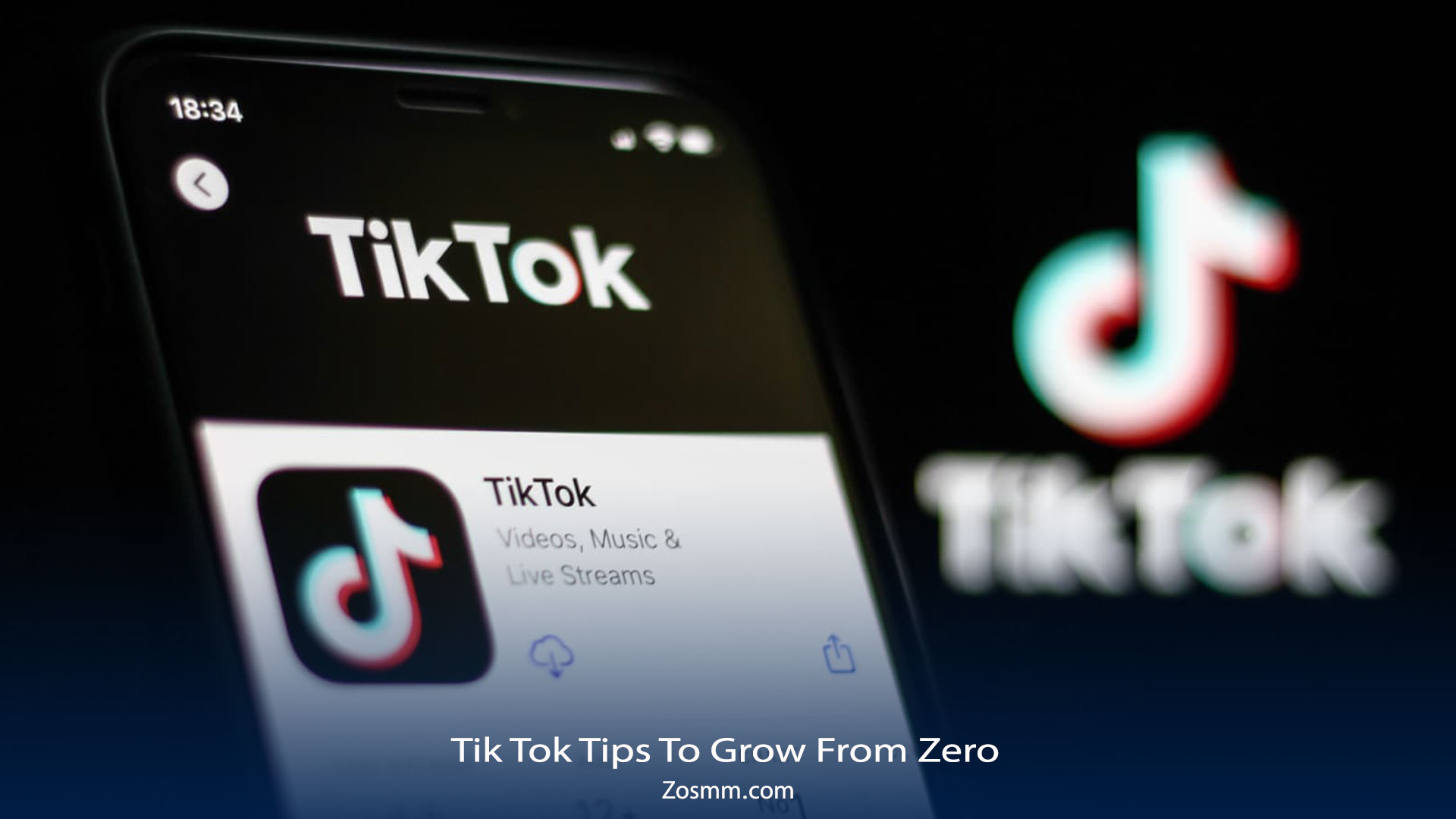This landscape-oriented image serves as an advertisement for a TikTok-related application or program, featuring a striking background that transitions seamlessly from black at the top to blue at the bottom. Dominating the foreground is a slightly angled smartphone with a black frame, presenting its vivid display. The screen shows the time "18:34" in white font at the top, along with somewhat blurry icons for battery, Wi-Fi, and another indistinguishable icon.

Beneath these details, a white circle with a left-pointing arrow and the "TikTok" name in its iconic font stand out against the black background. This section also displays a white box containing the TikTok logo, along with black text that reads, "TikTok video music and live streams." Nearby, the interface shows a cloud icon with a downward arrow, indicating a download button, alongside an upload button.

Further down, white text declares, "TikTok tips to grow from zero," followed by a website link, "zosmm.com." On the right side of the image, the TikTok logo appears again with a text overlay that creates a blurred effect, reinforcing the idea that this is indeed an advertisement. The intricate details and modern design elements effectively highlight the promotion of the TikTok-related app or program.